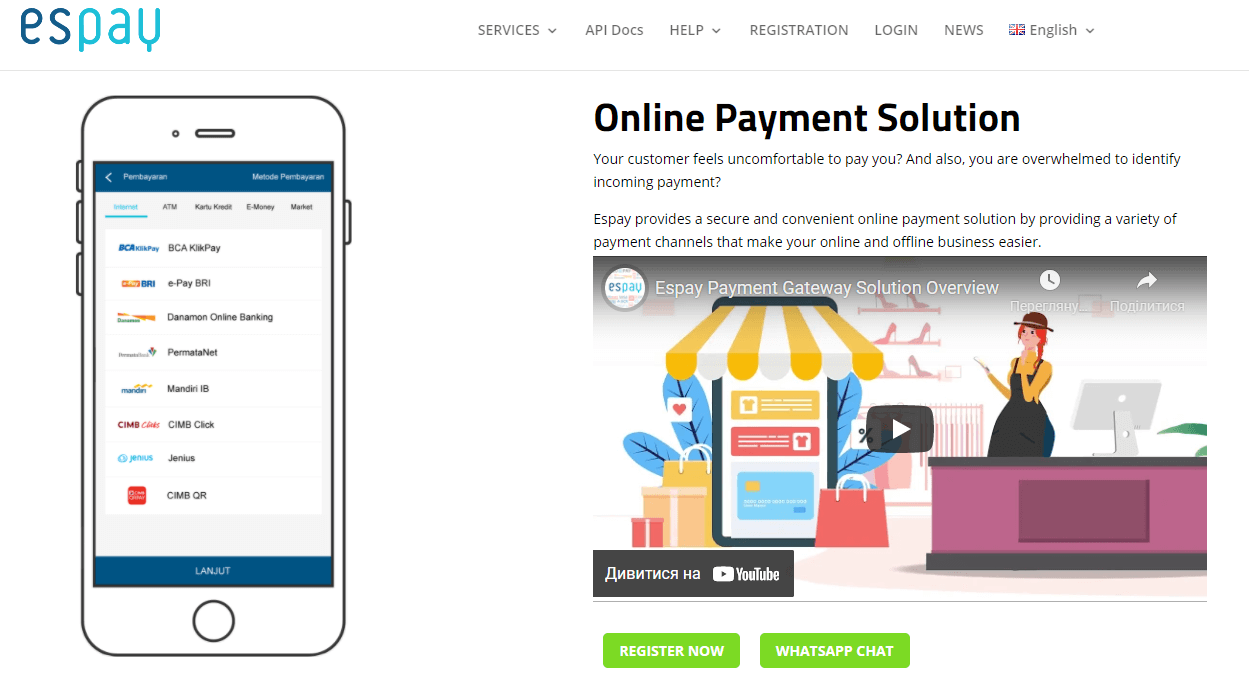In this image, the focal point is a white background with the word "SPAY" prominently displayed at the top. The page features a navigation bar that includes options for Services, API Docs, Help, Registration, Login, News, and language selection, set to English.

To the left of the image, there is a white smartphone with a blue highlight at the top. The phone screen displays a menu showcasing different brands, and a prominent white button is located at the bottom.

On the right side, text reads "Online Payment Solution," followed by a brief description of SPAY's services: "Your customer feels uncomfortable to pay you and also, you are overwhelmed to identify incoming payment. SPAY provides a secure and convenient online payment solution by offering a variety of payment channels that make your online and offline business easier."

Directly below this text is an illustrative graphic showing a circle with the SPAY logo inside it, alongside the heading “SPAY Payment Gateway Solution Overview.” Adding to the visual narrative, a woman stands behind a purple desk with a computer. Nearby, a small phone and several shopping bags are within the setup. 

In the bottom section of the image, there is a small black box labeled "Authentica" with a YouTube icon. Furthermore, two green buttons labeled "Register Now" and "WhatsApp Chat" are prominently displayed, encouraging user interaction.